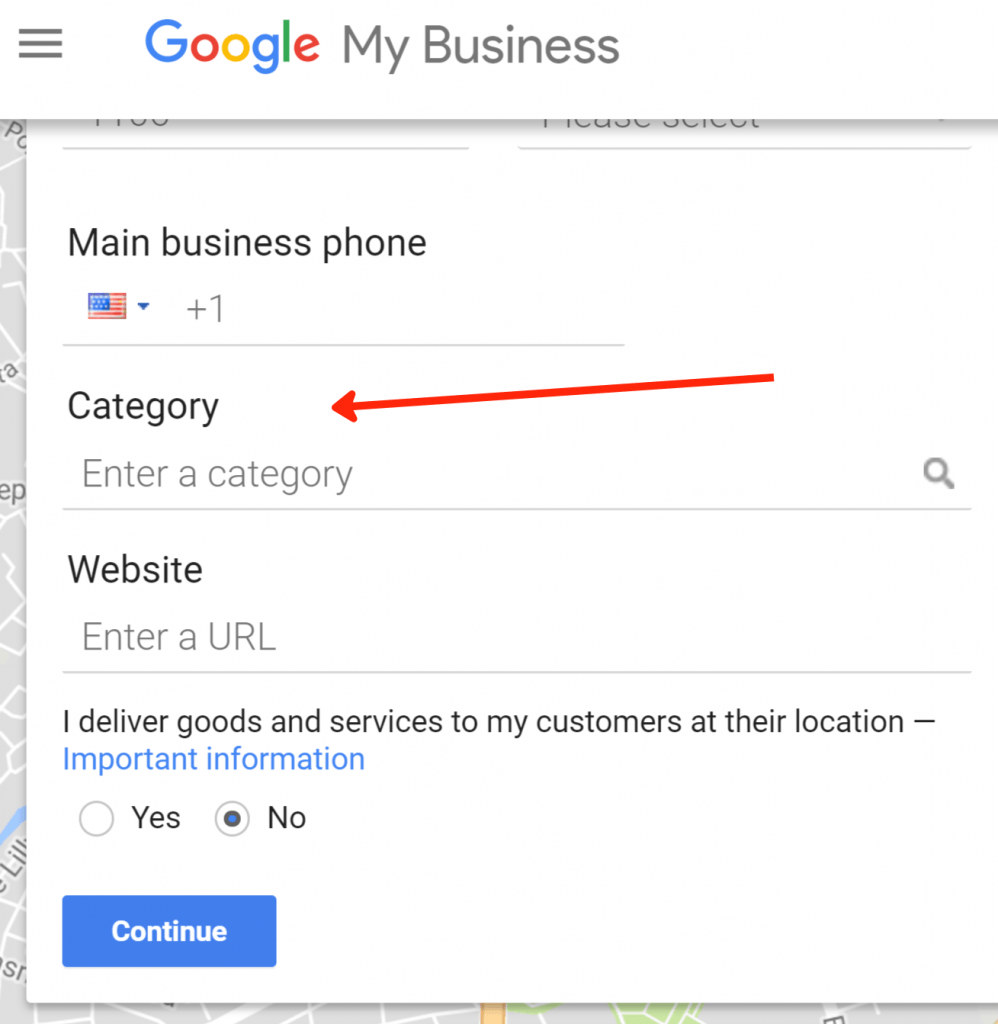The image depicts a person reviewing their Google My Business page. The interface shows the Google Maps background, partially obscured by a drop-down menu extending from a header with a significant drop shadow. In the header, a hamburger menu icon appears on the left, followed by the "Google My Business" logo where "My Business" is written in light gray font due to partial scrolling. The view is focused near the bottom of the tab, which reveals several input fields and options.

At the top, there’s a section labeled “Main Business phone” displaying the USA flag icon, followed by a “+1” country code and an underscore line for the phone number input. Below this, the word "category" is in bold, with an "enter a category" input box in darker text beside a magnifying glass search icon. A prominent red arrow points towards this category input field.

Further down, the word "website" appears in black text, with an "enter URL" input box aligned similarly to the category field but in gray text. Next, a statement reads, "I deliver goods and services to my customer at the location - import information" in blue text. Below this, a set of radio buttons presents the options "yes" and "no," with "no" currently selected.

At the bottom, there is a blue rectangular button with white text stating "Continue." The button appears to float above the map field beneath due to a drop shadow giving it a three-dimensional effect.